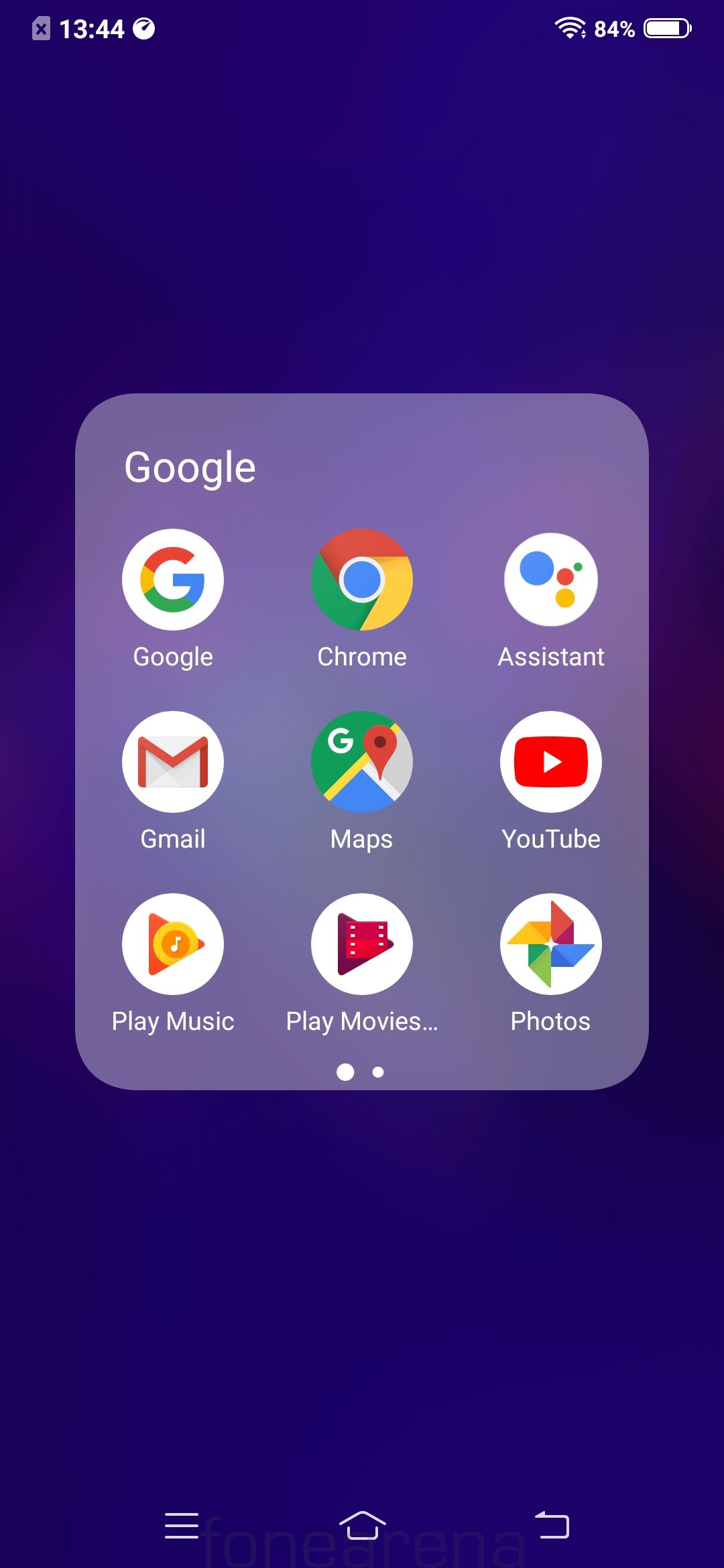The Android phone's homescreen is uniquely minimalistic, featuring a sole group folder labeled 'Google' rather than individual app icons. This folder contains several Google applications such as Google Chrome, Assistant, Gmail, Maps, YouTube, Play Music, Play Movies, and Photos, with additional apps accessible by scrolling, possibly including Drive and others. The background is a predominantly solid blue with subtle variations in lightness. The screen shows the battery at 84%, a strong Wi-Fi signal, and the time as 13:44. An icon indicates either no SIM card or an issue with SIM connectivity. At the bottom, there are three navigation buttons—back, home, and menu—reminiscent of older Android versions.